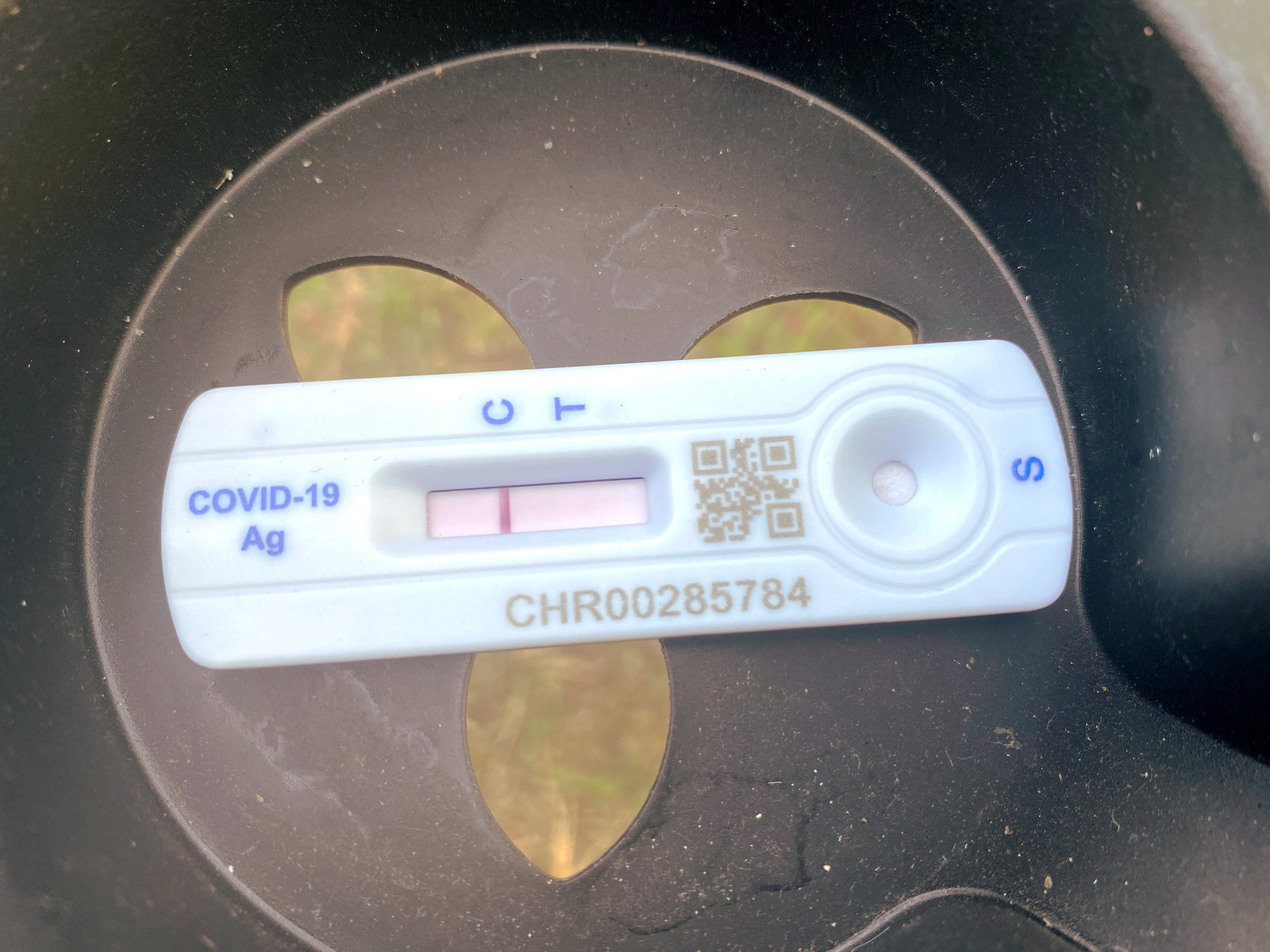A photograph captures a shiny black background that is both intriguing and peculiar, reminiscent of the inside of a muffin pan coated with a layer of dust, resembling dandruff or dander. This metal circular mold, commonly used for baking, features a central placement of a white plastic object that draws immediate attention. Surrounding this central object are four gold-like leaf shapes arranged in a trifoil pattern, adding a touch of elegance to the otherwise dusty appearance of the pan.

Centrally focused in the image is a white plastic COVID-19 test, positioned horizontally from left to right. The test’s exterior prominently displays "COVID-19" in blue font on the left side, with "AG" situated below it. At the top of the test, the letters "CT" are clearly marked in blue, while the bottom features a red font inscription: "CHR002835784." Adjacent to this text is a small QR code that can be scanned with a phone to access a website. A small white window embedded in the test reveals a single pink line, although it’s uncertain if this indicates a negative or positive result. This photograph juxtaposes elements of the mundane with the significance of contemporary health diagnostics, encapsulated within the dusty allure of a baking tool.